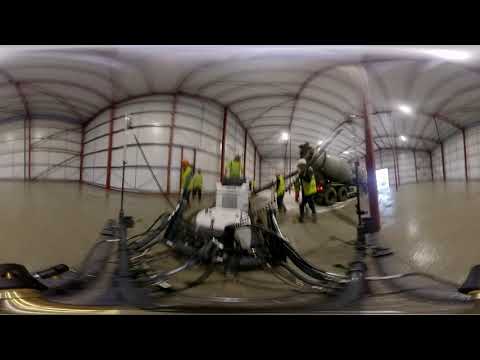The image depicts the interior of a large industrial-style building, possibly a warehouse, with a distorted 360-degree view. The structure features walls covered in white fabric or tarp, interspersed with thin red support beams and additional black beams. The ceiling has an arched design. Prominent in the image is a greenish concrete mixing truck positioned towards the right, actively pouring cement through an extension chute. Four to five men wearing yellow or highlighter green safety vests and jeans are working around the truck. Some are handling poles, likely to spread and smooth the freshly poured concrete, which appears shiny and dark in some areas, indicating it's still wet. Machinery can be seen at the front, including a white square object with multiple black cords. There are also two black pyramid-shaped objects with antennas, one in the center and a smaller one on the right. The floor in sections that have already been smoothed out contrasts with areas where the new cement has been poured. Despite the glare from the lights on the white walls, no windows are visible.